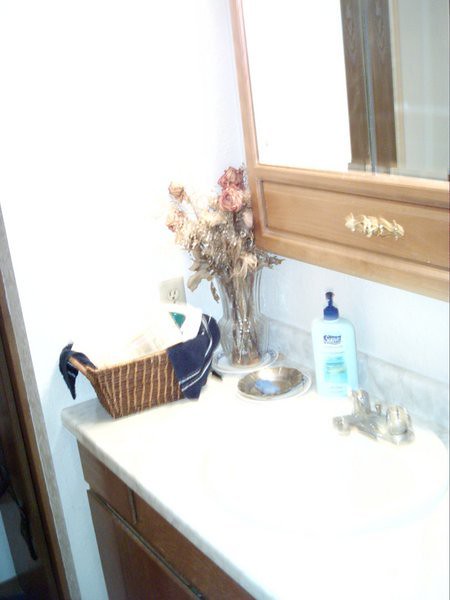The image depicts a somewhat blurry, old-fashioned bathroom that's not too antiquated but not entirely modern either. The camera angle is slightly downward, focusing mainly on the sink area. To the left, there's a doorway, and the wall appears white or possibly light blue, likely intensified by the camera's flash.

The sink is white, matching the countertop, which sits atop a wooden cabinet. Positioned to the far left of the sink is a basket containing something white, partially enveloped by a blue towel. Adjacent to the basket is a small bouquet of flowers, either fake or withering, showcasing hues of pink and red.

A bottle of Suave soap, characterized by its aqua color and blue cap, is placed near the flowers. The sink features silver fixtures. Above this setup, there is a wood-paneled mirror, although the right edge of it is not visible in the picture. The left side panel of the mirror is particularly thin, and the bottom border is adorned with intricate golden floral designs.